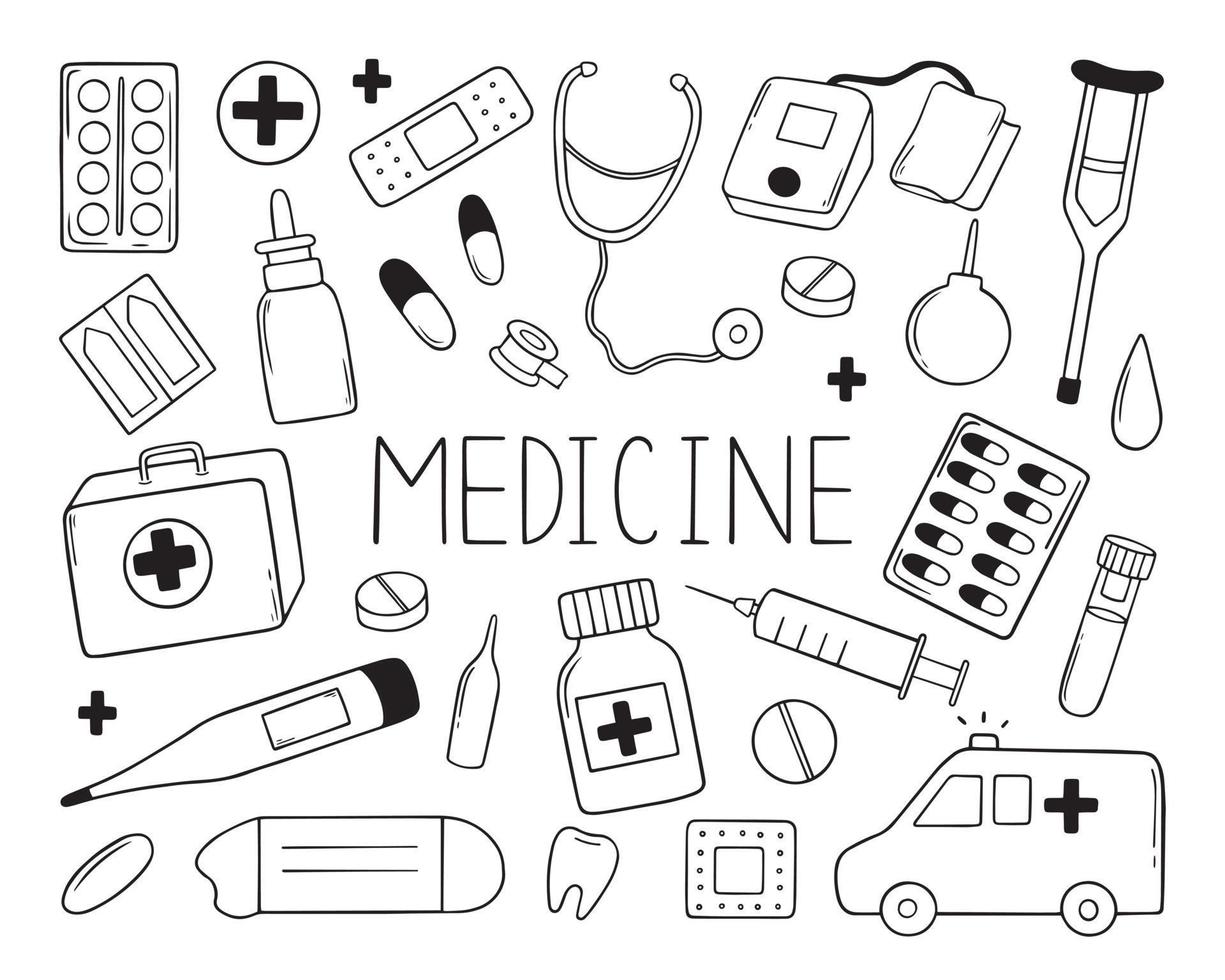The image is a detailed black-and-white illustration centered around the theme of medicine. At the heart of the image, the word "MEDICINE" is prominently displayed in large, black capital letters. Surrounding this central text are various outlined drawings of medical instruments and symbols. 

Above the word "MEDICINE," there is a drawing of a stethoscope. To the left, you can find outlines of a plaster, two tablets, a medicine bottle, two plus symbols, and another tablet. On the right side, the illustrations include a blood pressure machine, a crutch, and additional tablets. Below the central text, there is a medicine bottle marked with a plus sign. To the left of this bottle, the drawings depict a thermometer, a first aid box, and a tooth. To the right, there are images of a syringe, an ambulance, and a vial. 

This intricate collection of medical-related drawings showcases an array of equipment such as band-aids, blood pressure cuffs, pills, a flu shot needle, a dropper, and a test tube, all repetitively highlighting the essence of medical care and instruments.